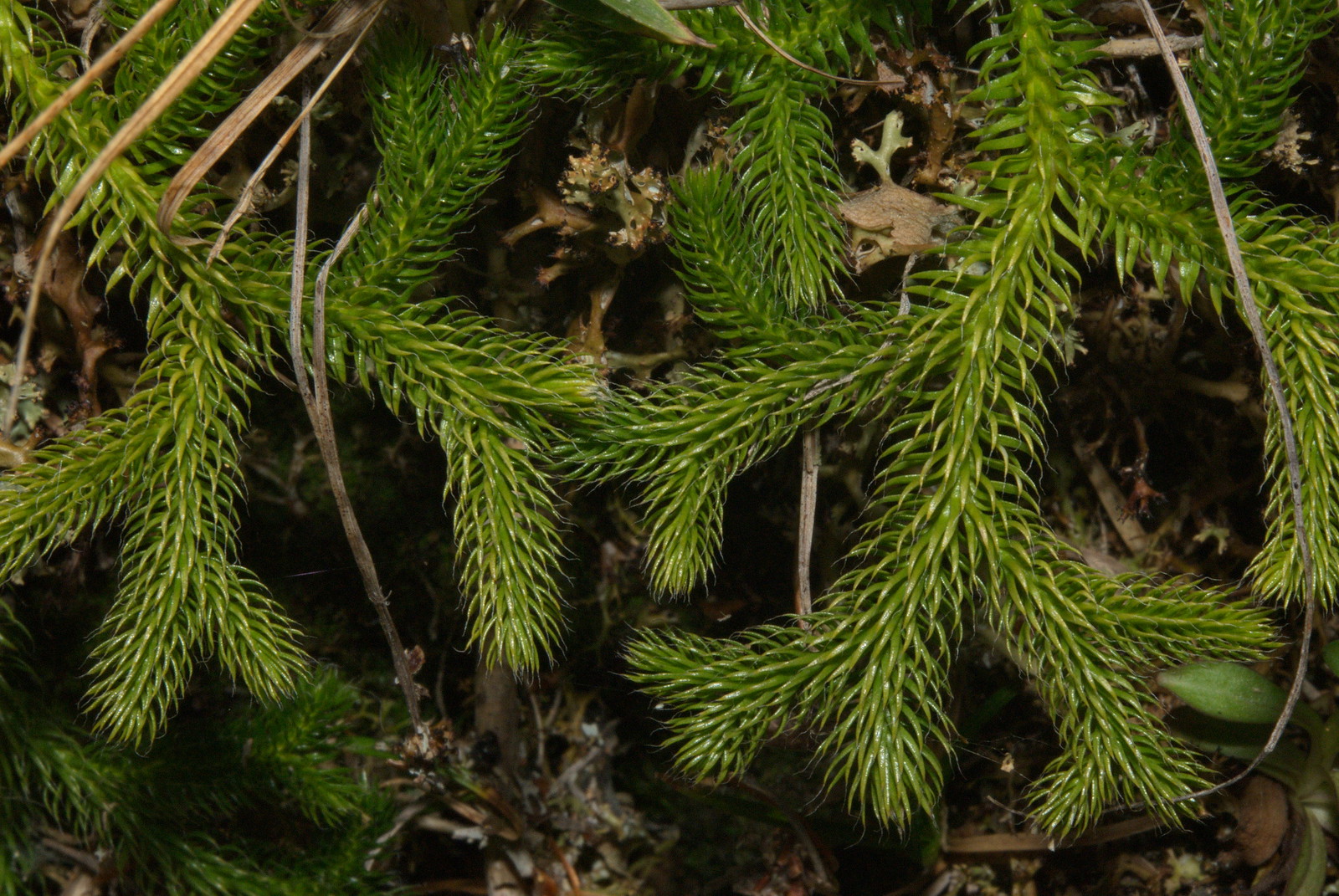This close-up image captures the intricate details of a branch from what appears to be an evergreen tree, possibly pine. The vibrant green needles are juxtaposed against a backdrop filled with a tangle of dry brown leaves, twigs, and dead vines. The needles, which look prickly and sharp enough to cause discomfort if touched, create a striking contrast against the myriad of browns and earth tones behind them. The texture and shininess of the needles are so pronounced that they almost appear artificial, suggesting a high level of detail in the photograph. This detailed depiction leaves viewers contemplating whether the setting is indoors or outdoors, potentially resembling a Christmas wreath with its complex blend of green and woody elements.